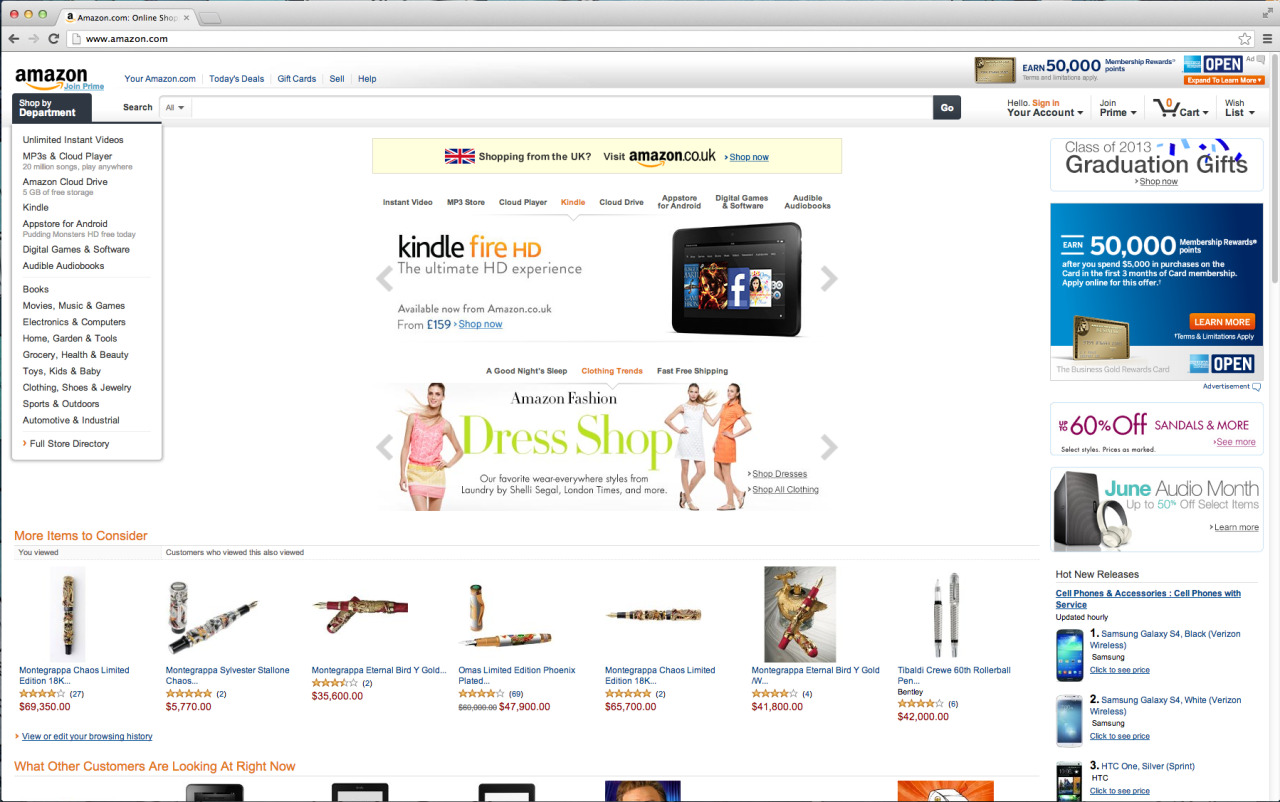This image is a screenshot of an older version of the Amazon.com website. The top of the page includes a notification prompting users shopping from the UK to visit Amazon.co.uk, with a direct link provided. Additionally, there's a prominent search bar displayed at the top center.

On the left side of the page, a menu features various departments under the heading "Shop by Department." These categories include:

- Unlimited Instant Videos
- MP3s and Cloud Player
- Amazon Cloud Drive
- Kindle
- App Store for Android
- Digital Games and Software
- Audible Audiobooks

Further down, more traditional product categories are listed, such as:

- Books, Movies, Music, and Games
- Electronics and Computers
- Home, Garden, and Tools
- Grocery, Health, and Beauty
- Toys, Kids, and Baby
- Clothing, Shoes, and Jewelry
- Sports and Outdoors
- Automotive and Industrial

At the bottom of this menu, there is a link to a "Full Store Directory" for users seeking more specific sections.

The main body of the page features various advertisements. Prominent ads include promotions for Amazon Fashion and the Kindle Fire HD. Other advertisements highlight deals from different companies, such as "60% Off Sandals" and "June Audio Month."

Toward the very bottom of the screenshot, several listings for different types of fountain pens are visible, showcasing a variety of options available for purchase.